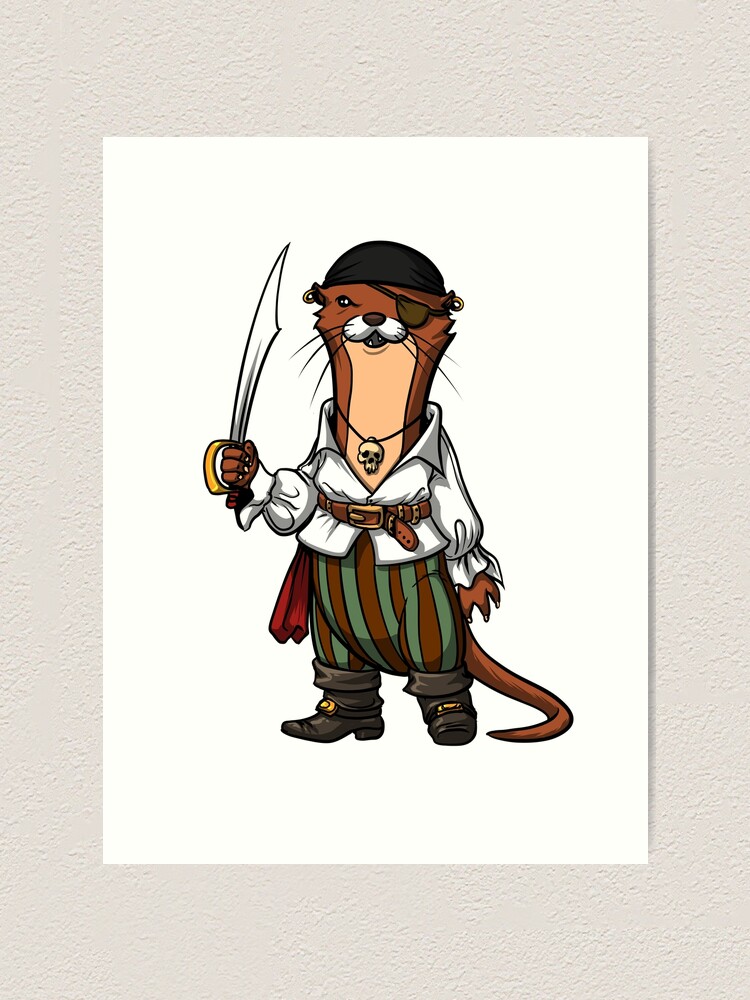The illustration presented on a white canvas with a large cream border depicts a cartoonish, anthropomorphic otter dressed as a pirate. The otter stands upright on its hind legs with brown fur and a beige chest. It wears a black hat and an eye patch over its left eye, accessorized with tiny gold hoop earrings. Around its long neck hangs a black skull necklace. The otter is clad in a classic pirate ensemble featuring a frilly, puffy white pirate shirt belted at the waist with a brown belt, accompanied by red and green vertically striped pants. Its black boots feature prominent gold buckles. The otter's left hand grips a scimitar with the blade pointed upwards, while a red sash adorns its side. Its tail curls noticeably towards the right side, adding a playful touch to the depiction.